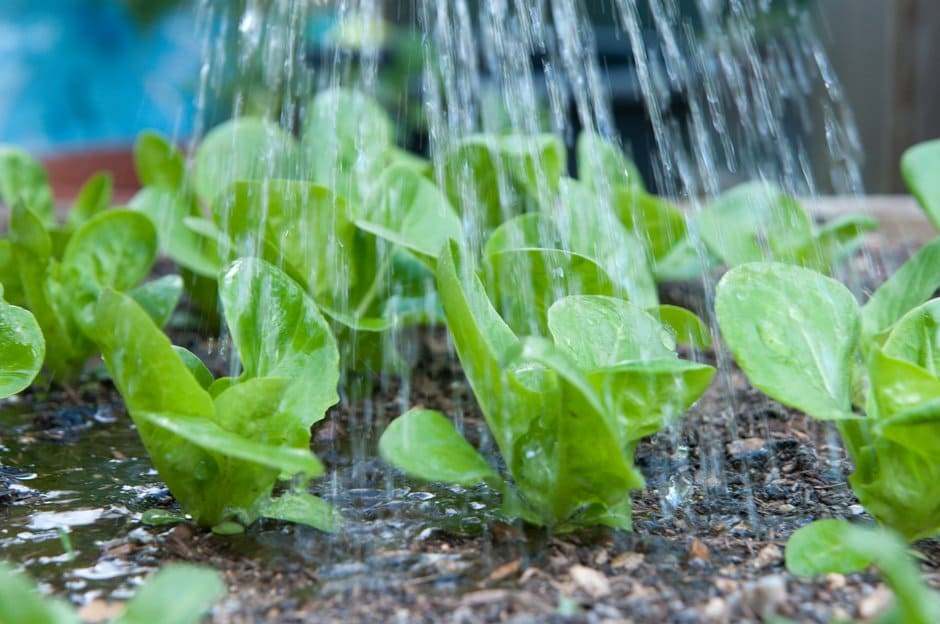This photograph features a group of approximately 25 very young green plants, likely lettuce seedlings, being showered with water from above. The water cascades down, hitting both the tiny, vein-marked leaves and the uniformly brown soil, with some areas already wet and others still dry as the watering has just begun. The scene captures droplets scattering in a raindrop-like pattern, creating a freshly watered, muddy patch of ground. The plants, nestled in a reddish terracotta pot or raised planter, fill the entire frame, while a blurry background reveals a bright cerulean blue and terracotta red, possibly other pots or elements. The source of the water, possibly a hose sprayer, remains off-frame, but the impact on the plants is clear with their wet, vibrant green leaves standing out against the dark, damp earth.